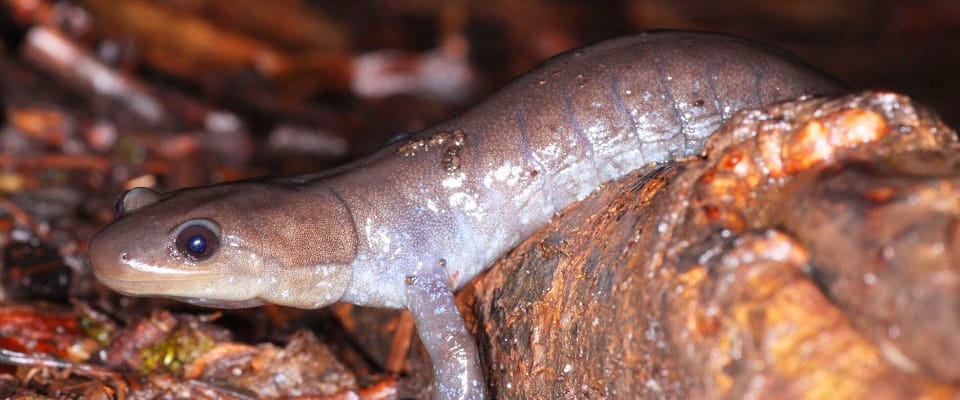The detailed image depicts a lizard, or possibly a salamander, in a close-up, naturalistic setting. The lizard's smooth body features a brown color on top, transitioning into a yellow gradient near its head and a gray gradient along its body toward its paler underbelly. It has pronounced, human-like brown eyes with visible sclera. The lizard's head is positioned on the left side of the picture, while its body arches upward as it traverses a log or tree root, which takes up space towards the right-hand side of the image. The surrounding environment consists of wet leaves, sticks, and muted colors, including various shades of brown, gray, black, white, with hints of orange and red, suggesting a forest or jungle floor, although it could also be an artificially crafted habitat. The overall setting hints at a wetland or rainforest ambiance, and despite the placement of the lizard's body towards the center and top of the screen, its tail is not visible in the image.